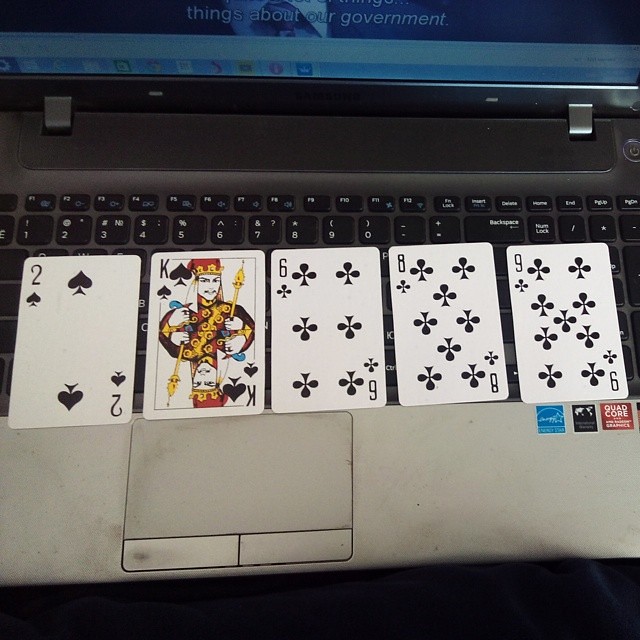This image captures the detailed view of an open laptop. The focus is on the keyboard and touchpad area. The bottom portion of the laptop, finished in a sleek silver tone, houses the touchpad with separate left and right mouse buttons. Just above this silver section, the keyboard area is composed of a darker gray plastic adorned with black keys featuring white lettering.

On the far right corner of the silver section, three logo stickers are visible: one in blue from Intel, and two others in black and red, though their exact labels are indistinguishable.

Spanning the keyboard from left to right are four playing cards laid out face-up: the two of spades, the king of spades, the six of clubs, and the eight and nine of clubs, all depicted in black.

Only the upper quarter of the image reveals a portion of the laptop's monitor. A faint gray-blue line runs horizontally across the top, beneath which a segment of the screen shows text with white lettering, discussing matters related to the government.